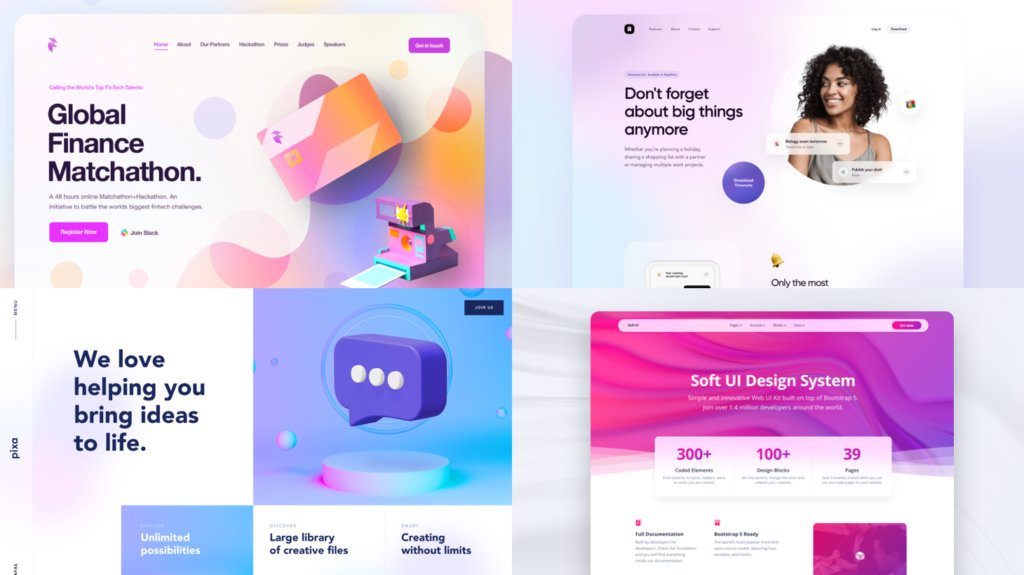The image is a screenshot depicting a design system and global finance theme, divided into four distinct sections, arranged in a 2x2 grid format.

* **Top Left Box**: Titled "Global Finance Matchathon," this section features a vibrant design in shades of orange, pink, and blue. At its center is a Polaroid camera, from which a photo is emerging. The background is adorned with small colorful circles in hues of purple, orange, and pink, creating a dynamic visual effect.
  
* **Top Right Box**: This section bears the title "Don't Forget About Big Things Anymore." On the right side, there is an image of a smiling, dark-skinned woman with almost shoulder-length dark hair. She is looking to the left and is dressed in a gray sleeveless top. The box also includes a prominent purple circle at the center, although the accompanying text is too small to discern.
  
* **Bottom Left Box**: Marked by the headline "We Love Helping You Bring Ideas to Life," this area includes a purple speech bubble containing three white dots, positioned over a white circular object. The background is blue with a circle framing the speech bubble. At the bottom of the box, there are additional statements: "Unlimited Possibilities," "Large Library of Creative Files," and "Creating Without Limits."
  
* **Bottom Right Box**: This portion is decorated with a swirling purple and dark pink design at the top and is labeled "Soft UI Design System" in the center. The rest of the text in this box remains too small to read.

Overall, the screenshot presents a colorful and harmonious layout, rich in visuals and varied design elements that collectively emphasize themes of creativity and innovation in global finance and design systems.